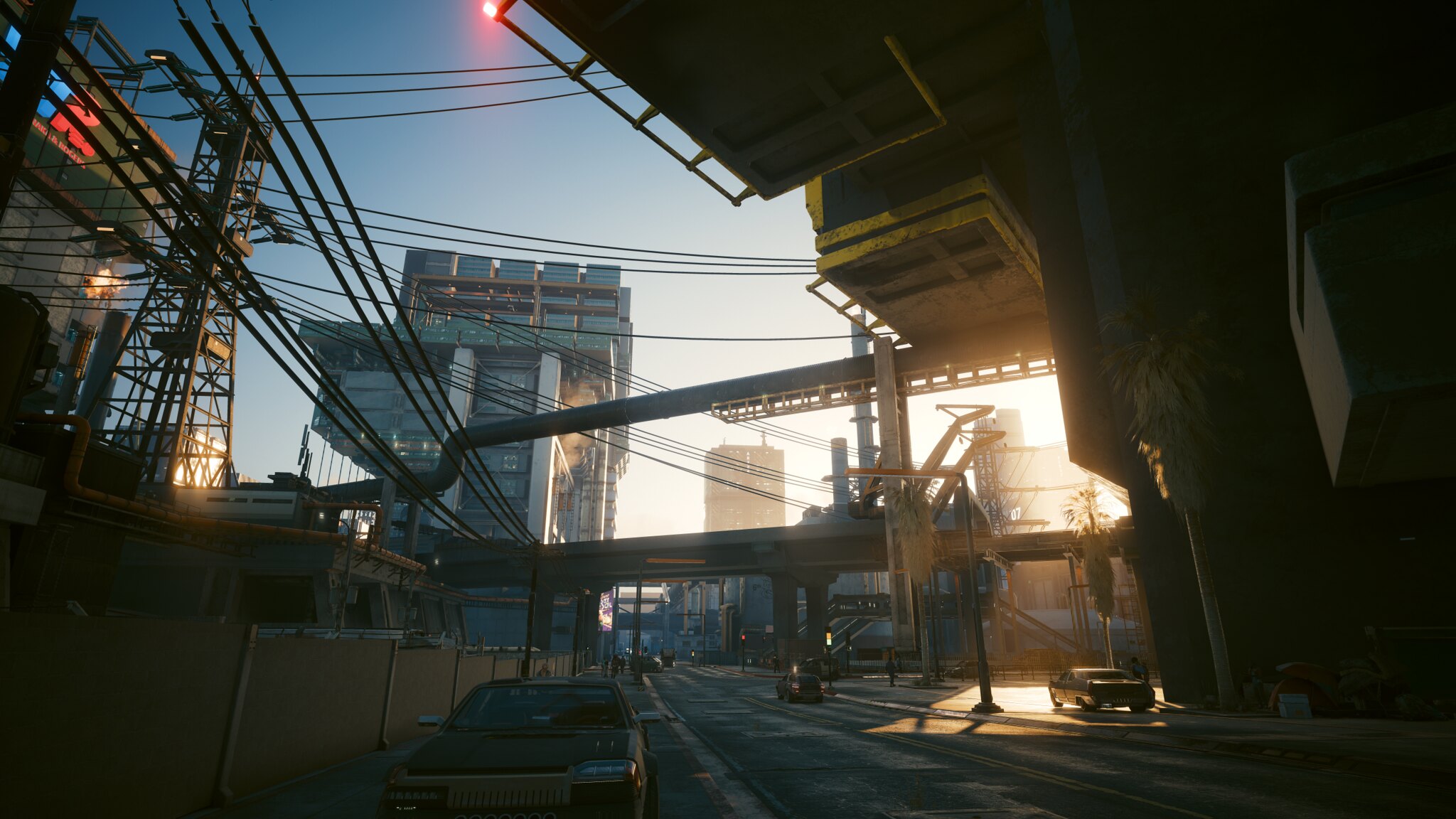In this intricate and bustling industrial scene, a towering building dominates the background, exemplifying the imposing infrastructure of the area. To the right, a vast raised walkway or possibly an elevated structure with a prominent yellow section juts out, casting its shadow below. The image is a web of activity, with various pipes, cables, and bridges crisscrossing throughout, many of which are supported by robust pillars. In the cluttered foreground, a car is parked towards the left, partially obscured by a wall or fence and surrounded by numerous girders. Adding a splash of vividness, a bright red 'A' is prominently displayed near the top of a building on the left, drawing the eye amid the industrial chaos.